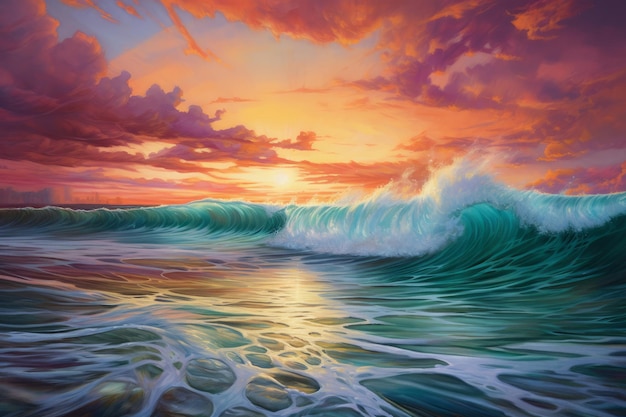This image showcases a handcrafted or digital painting illustrating a serene oceanic scene. The centerpiece of the artwork portrays waves crashing with vivid realism, creating foamy textures in the foreground. The ocean is depicted in a spectrum of blues, teals, and light greens, highlighting the dynamic movement of the water. Above, an amber-hued sky with deep pink and orange-tinted clouds complements the setting sun. The sun, positioned centrally, emits a bright white reflection across the water’s surface, enhancing the tranquil ambiance. The sky darkens progressively towards the top and corners of the image, emphasizing the diminishing daylight. The composition is balanced, with the ocean dominating the lower half and the sky occupying the upper half, drawing the viewer's attention to the harmonious interplay of natural elements in this outdoor scene.